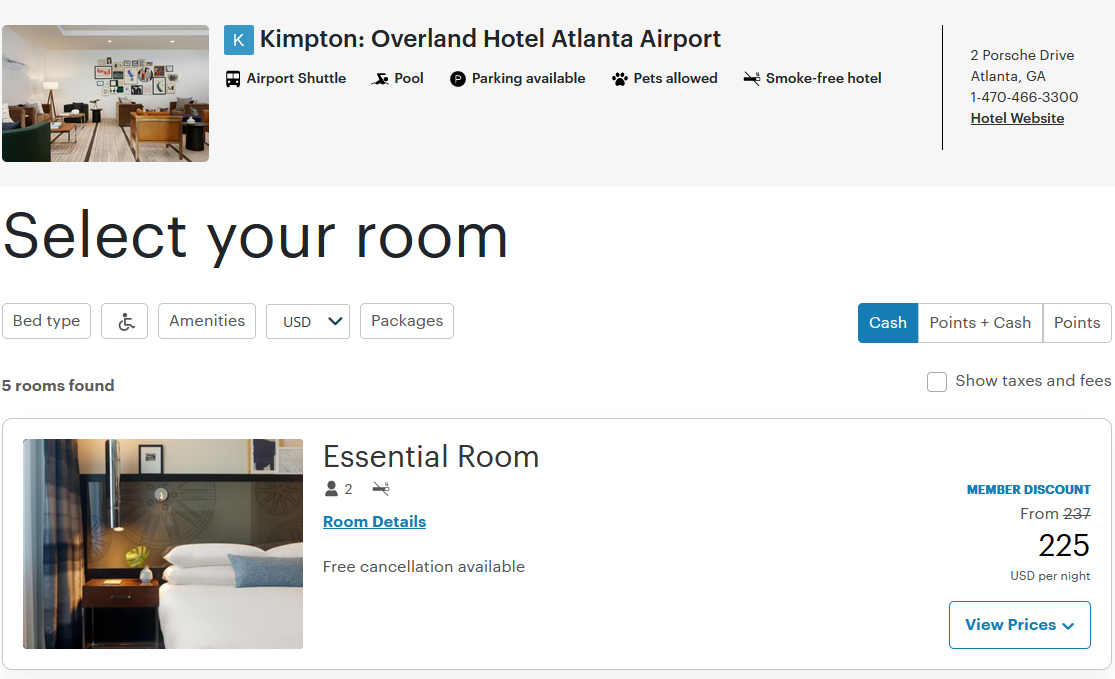This is a detailed screenshot of a website featuring information about the Kempton Overland Hotel Atlanta Airport. At the top, there is a gray rectangle. On the left side of this rectangle, there is a small photo of a cluttered white room, showcasing a couch, a table, and numerous photos arranged on the wall. To the right of the photo, the hotel name is displayed: "Kempton: Overland Hotel Atlanta Airport." Adjacent to the hotel's name on the left is a blue square with a white 'K' in it. Below the hotel name, a list of amenities is provided: "Airport Shuttle, Pool, Parking Available, Pets Allowed, Smoke-Free Hotel."

To the right of the amenities list, the hotel's address and contact information are displayed: "2 Porsche Drive, Atlanta, Georgia, 1-470-466-3300," followed by a link to the hotel website. Below this, in a white rectangle, the website prompts users to "Select Your Room Bed Type." Icons indicating accessibility features, such as a person in a wheelchair, are shown alongside options for amenities and payment methods, the latter of which includes USD, Points, and Cash; the option "Cash" is currently selected. Further down is a clickable white square labeled "Show Taxes and Fees," and a note indicating that "5 rooms found" completes the information shown.